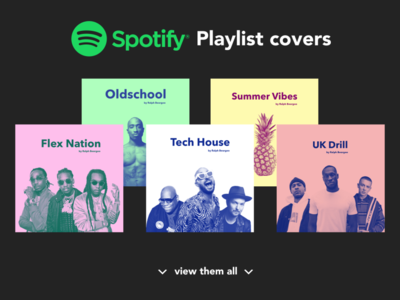This is a detailed advertisement for Spotify. The primary features include a black background with a small black rectangle, featuring a green circle hosting three black lines—Spotify's iconic logo. Adjacent to the logo, the text "Spotify" is displayed, followed by a barely visible trademark symbol due to its diminutive size.

Next to the logo text, a prominent white text declares "Playlist Covers." Below this heading lie five album covers arranged prominently:

1. **Flex Nation**: The cover showcases three African-American men, all dressed in shirts. The central figure sports a jacket, and all wear watches. The man on the right has braids, while the man on the left has his hair pulled back into a ponytail or man bun. The album title "Flex Nation" is in bold, with smaller, difficult-to-read text underneath.
   
2. **Tech House**: This cover features one African-American male and two white males. Notably, one of the white males is bald, the other dons a hat, and wacky glasses atop a vibrant, patterned shirt. The African-American male also wears glasses and is bald.

3. **UK Drill**: This cover has three men: the one on the left may be Latino, the middle man is African-American, and the man on the right is white.

Behind these three album covers are two staggered, partially concealed album covers:

4. **Old School**: Positioned slightly behind "Flex Nation" and "Tech House," this cover is green with blue text. It prominently features an image that might be Tupac, peeking between the albums in front.

5. **Summer Vibes**: This cover is yellow with a pineapple illustration and the text "Summer Vibes." It is partially visible behind "UK Drill" and "Tech House."

At the bottom of the advertisement, a white drop-down arrow points downward beside the text "View Them All," suggesting more content can be accessed by clicking or tapping the arrow.